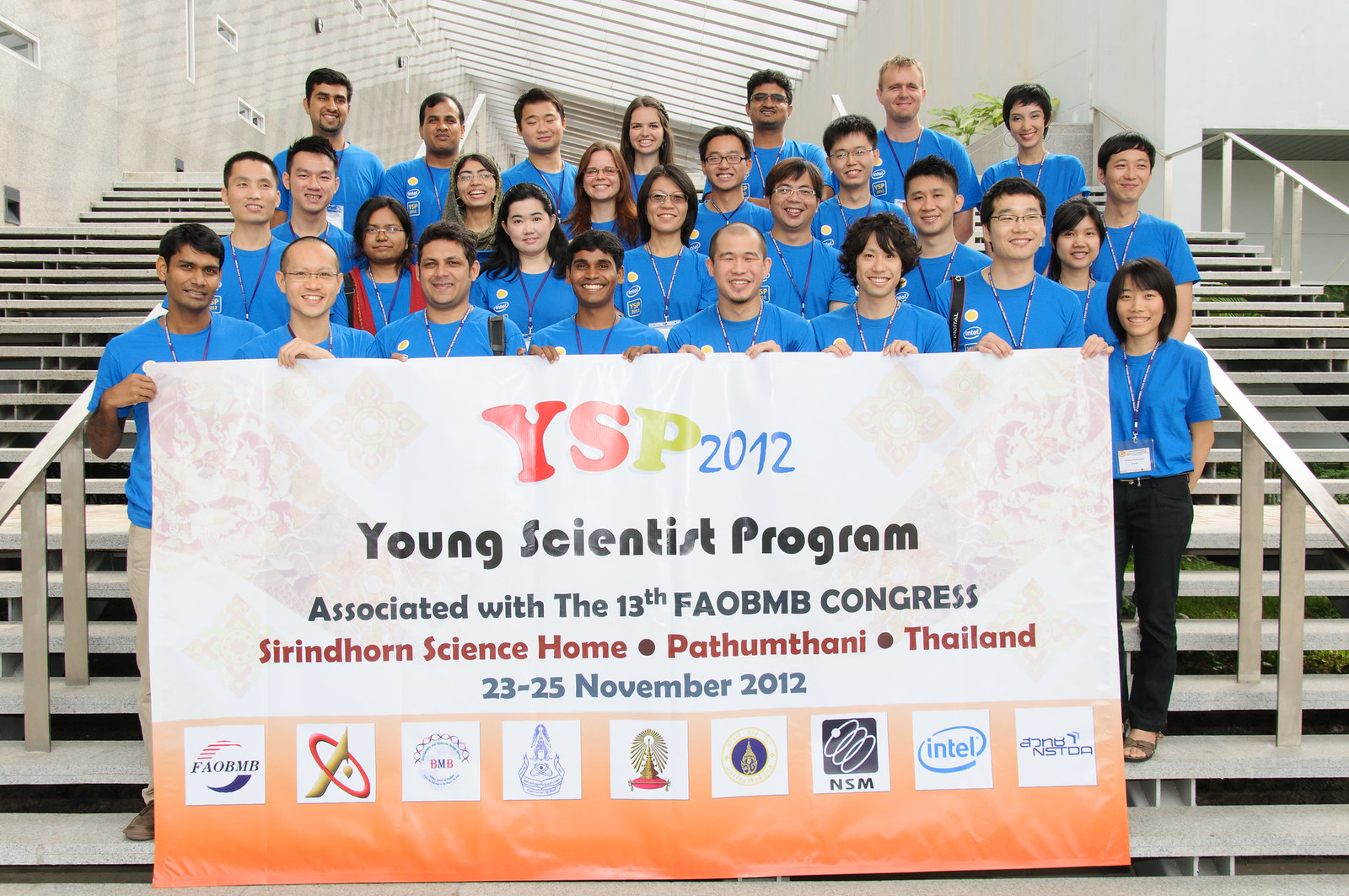The photograph is a wide rectangular image capturing a diverse group of young students, predominantly of Asian descent with some individuals of Caucasian and South Asian lineage, standing on a tall and wide stairwell in front of a light stone-colored building. The structure features an open-air space with an arched roof. Each of the students, estimated to be aged between 18 to 22, wears a blue short-sleeved T-shirt and has a lanyard, likely with a name tag, around their neck. The students are organized into four rows on the staircase, with the front row of nine students holding a large white and orange banner. The banner displays "YSP 2012" in colorful letters, with the 'Y' in red, 'S' in orange, and 'P' in green. Below this, in black print, it reads "Young Scientist Program associated with the 13th FAOBNB Congress." Further down, in red and blue, it states, "Sirindhorn Science Home, Pathumthani, Thailand" and the dates "23-25 November 2012." The banner also features an orange footer adorned with various sponsor logos, including one from Intel. The building in the background, with its elegant design, gives the impression of an academic institution.